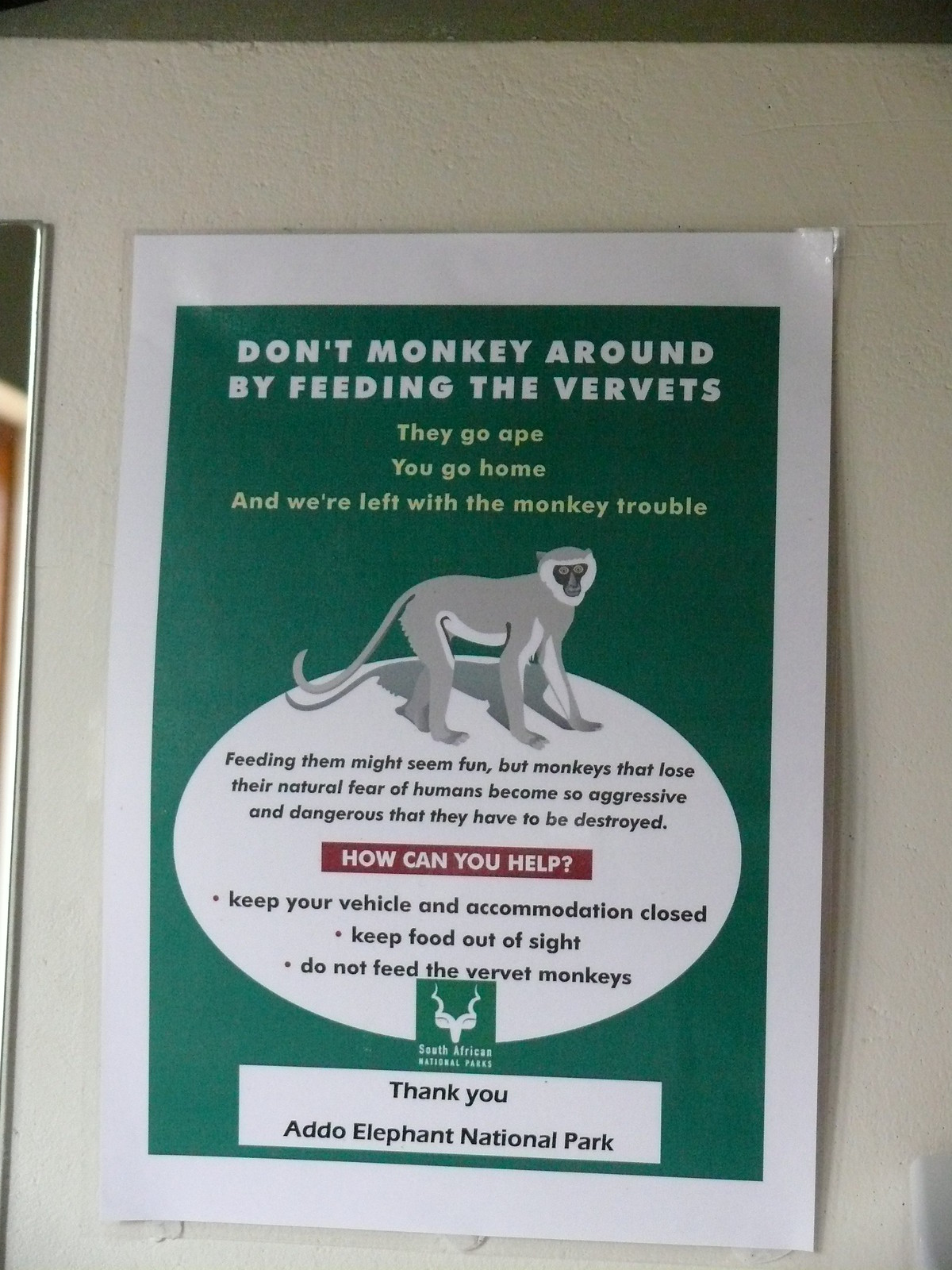Displayed on a white wall, a laminated poster with a white border and a green background delivers an urgent message. The central message, in bold white text, reads: "Don't monkey around by feeding the vervets. They go ape. You go home, and we're left with monkey trouble." Below this, a detailed paragraph explains that "Feeding them might seem fun, but monkeys that lose their natural fear of humans become so aggressive and dangerous that they have to be destroyed." A grey monkey with a long tail faces the right side of the poster, providing a stark visual reminder. Towards the bottom, a red box titled "How Can You Help?" lists three bullet points: "Keep your vehicle and accommodations closed," "Keep food out of sight," and "Do not feed the vervet monkeys." The poster is signed off by Addo Elephant National Park and is affixed to the wall using a putty-like substance.